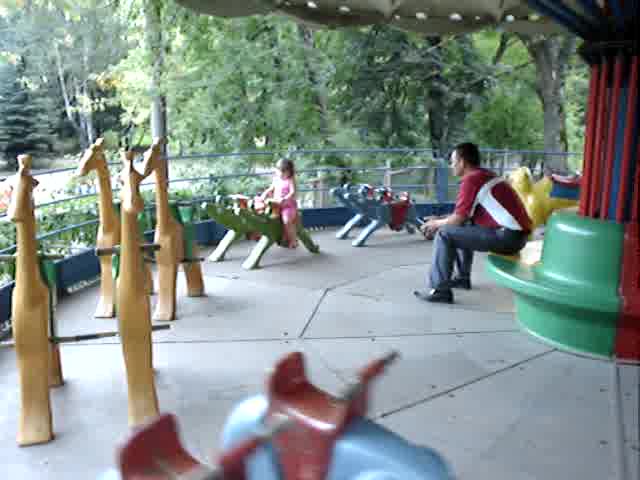In this slightly blurry square photograph, the scene is set outdoors at what appears to be a stationary carousel in the middle of the day. The central figure is an adult man who is seated on a round green bench, integrated into the carousel’s central column. He is dressed in a red and white short-sleeve shirt with grey pants and black shoes. The man gazes at a little girl wearing a pink outfit and sporting brown bangs, who is positioned on top of a carousel animal, which could potentially be a small horse or dog. 

Surrounding the girl, four golden yellow giraffe figures can be seen, and further ahead, there are two vibrant blue carousel animals adorned with red saddles. Directly behind her, another pair of blue creatures, also with red saddles, are visible. The background reveals a stand of lush green trees and a three-rail fence encircling the carousel. The ground appears to be made of a hard, gray stone surface, adding to the setting’s outdoor ambiance. The color palette of the photograph includes shades of red, blue, green, yellow, gray, and maroon, all contributing to the lively yet tranquil atmosphere of this moment captured at a possibly idle carnival carousel.